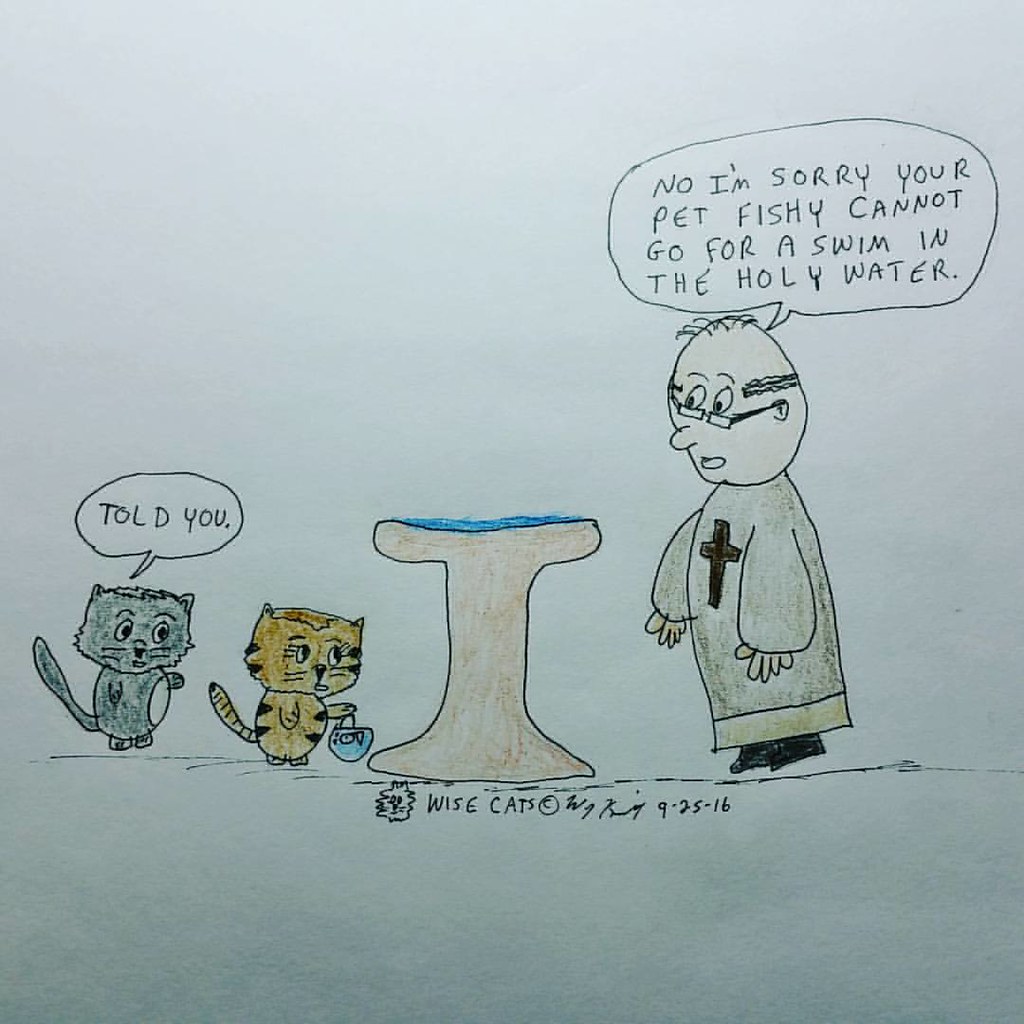This is a detailed, hand-drawn image printed on white paper, featuring two cats on the left and a man on the right. The first cat is grey with a white belly, and the second cat is orange with black stripes, holding a small blue bucket. The man, identifiable as a priest due to his attire, has thinning hair on top and glasses. He is depicted in a grey and gold gown with a cross on it, and black shoes. The priest is reaching out with his right hand, saying in a speech bubble, "No, I'm sorry, your pet fishy cannot go for a swim in the holy water." The grey cat responds with "Told you," also in a speech bubble. The background includes a holy water fountain, colored in brown and tan, near which the scene unfolds. The overall colors featured in the image are brown, tan, white, gray, and blue. The artist has signed and dated the drawing, with the signature reading "9-25-16." Additional text at the bottom of the image reads "Wise cats."